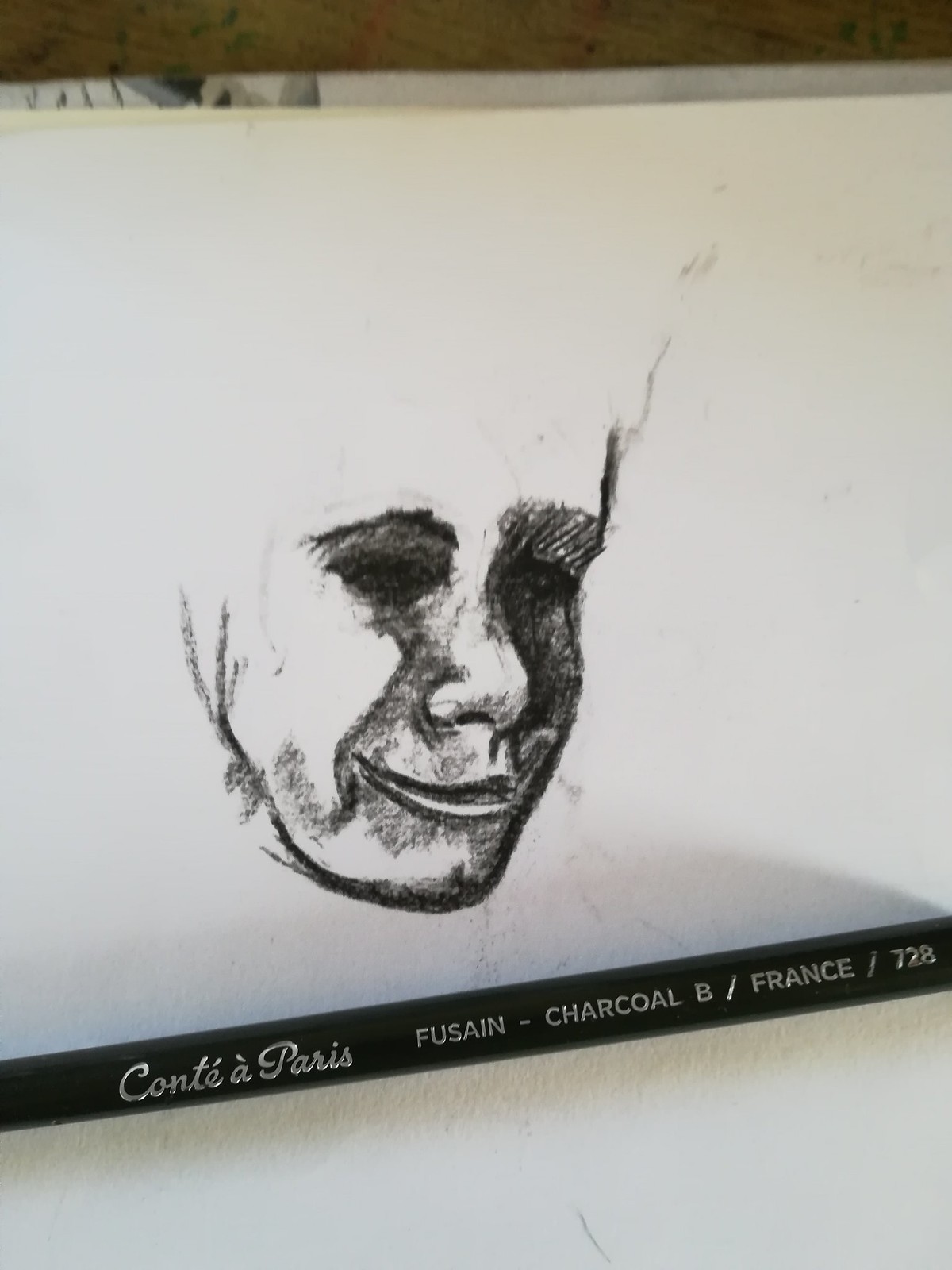This is a detailed black-and-white sketch of a person's face, centrally positioned on a piece of white paper. The face, depicted in profile, is oriented towards the right side of the image. Distinct facial features such as the eyes (represented as solid black), nose, mouth, and cheek are clearly illustrated, while the ears and hair are not visible. At the bottom of the image, there is a black pencil inscribed with the text "CONTE A Paris" on its side.